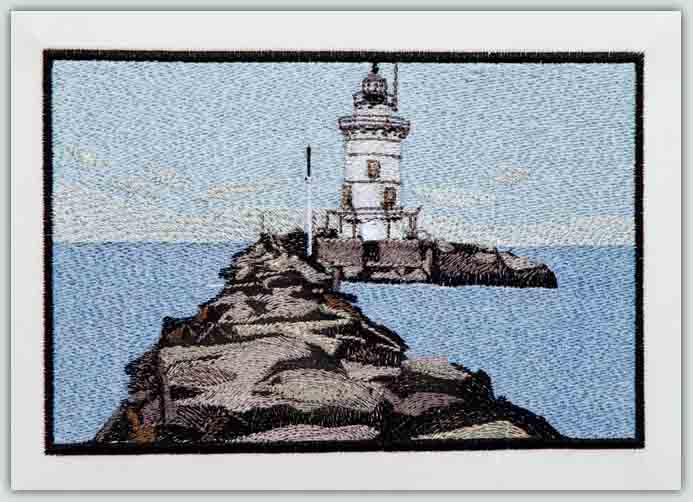This contemporary artwork depicts a white lighthouse perched on dark gray and black rocks, extending from the immediate foreground into the distance. An elevated rocky pathway leads to the lighthouse, framed by a body of deep navy blue water to the side. The sky above is a light blue, creating a serene backdrop. The entire image appears to be rendered in an intricate, embroidered-like style, with the details meticulously crafted to resemble tiny threads and flecks. The piece is bordered by a black frame, encased within a thicker white border, adding to its modern yet classic aesthetic.